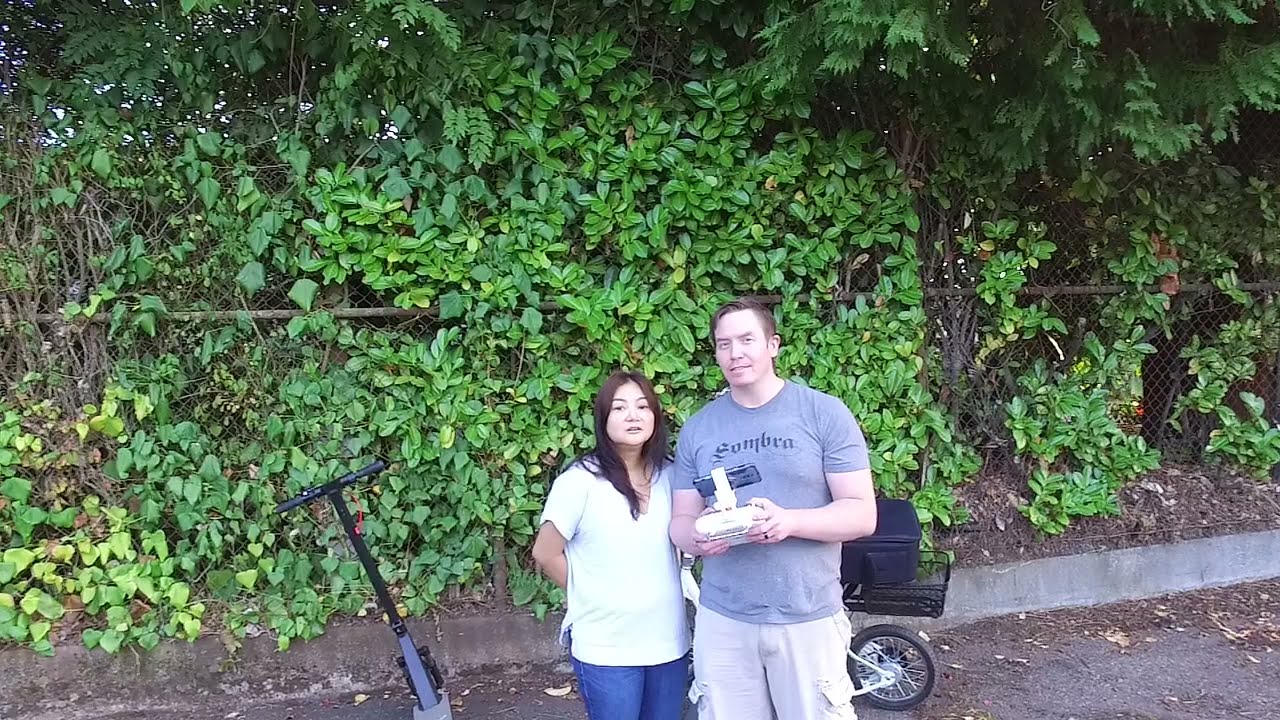This color photograph captures a couple posing on a leafy path, with an urban backdrop. The woman, of Asian descent, stands to the left, dressed in a white blouse and denim jeans. Beside her is an electric scooter. The man, a white guy, stands to the right in a gray t-shirt with black text, khaki cargo shorts, and holds what appears to be a drone controller with his phone attached. Behind them, a chain-link fence overgrown with vegetation and trees frames the scene. The path is paved with asphalt, scattered with brown plant debris. An electric bike is also visible behind the man. The setting is a blend of nature and urban elements, enhancing the coziness and casualness of the moment.